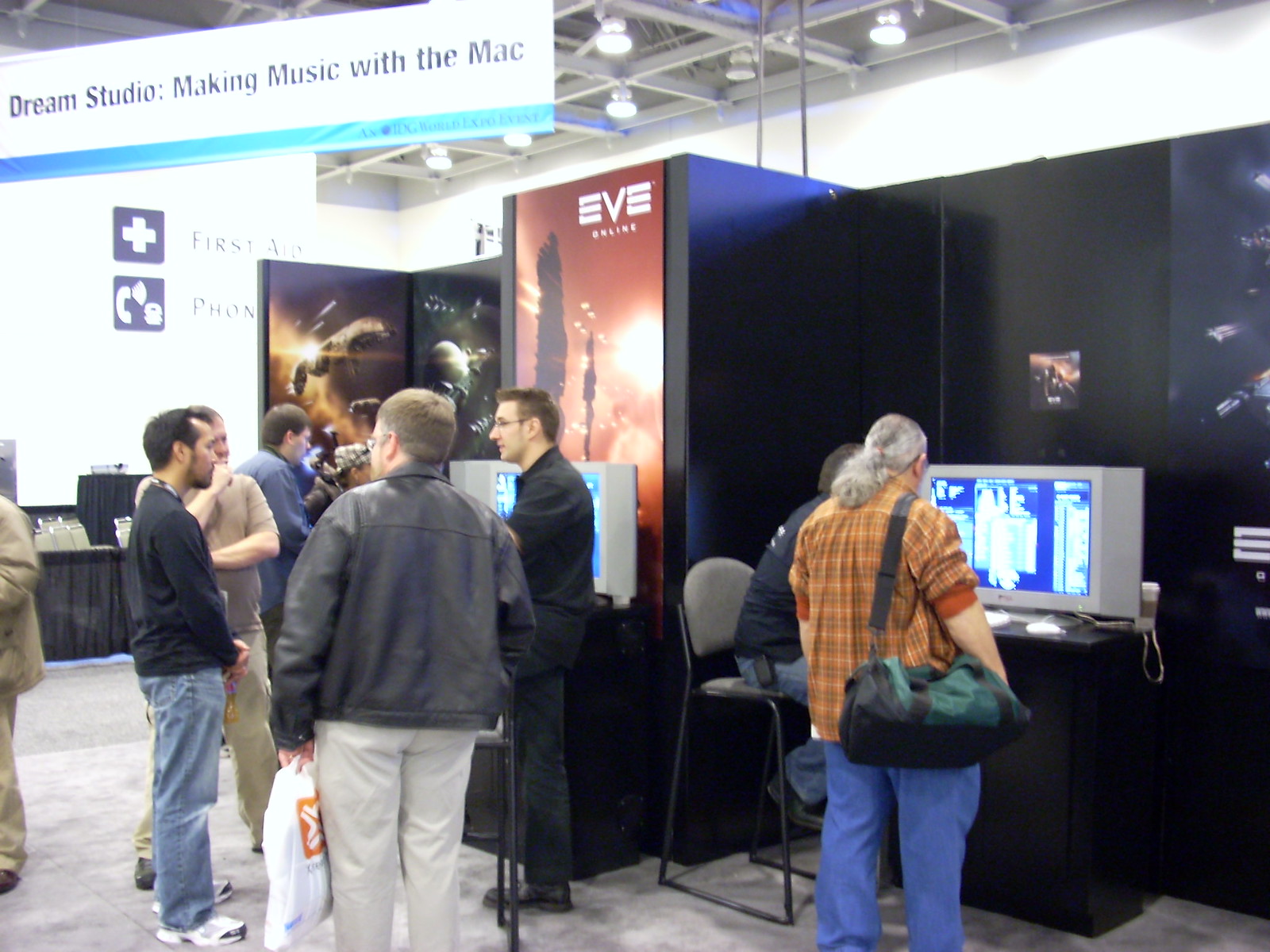In this image, we see an indoor setting that appears to be some kind of tech convention, taking place on a tile floor. The scene features several individuals, predominantly men, standing in the center and engaged in conversation. They are surrounded by various displays and tables covered with black tablecloths. Off to the right, there is a computer display with large screens and keyboards. At the top of the image, a prominent sign reads "Dream Studio, making music with the Mac," featuring a white background, black font, and a green stripe. The warehouse-like ceiling is outfitted with metal posts forming square patterns, each containing white lights. In the background, the white wall features various posters including one with the word "Eve" on an orange background and others displaying techie-type or outer space themes. The overall ambience is illuminated by the ceiling lights, adding to the bustling, high-tech atmosphere of the convention.